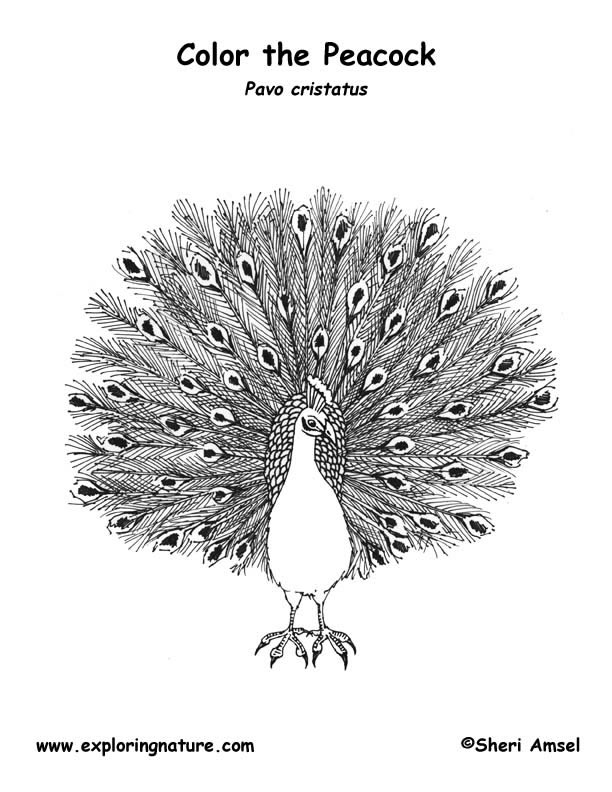This image depicts a detailed black and white coloring page focused on a male peacock with its feathers fully spread. The intricate illustration, executed in a sketchy, scratchy style, occupies the center of the page. The peacock's body faces forward while its head tilts slightly downwards to the left. At the top of the page, the words "Color the Peacock" are centered in Comic Sans font, followed by the scientific name of the species, "Pavo cristatus," italicized beneath it. The entire artwork, including text, is rendered in black on a white background. Below the peacock, the URL "www.exploringnature.com" is printed on the left, and the name "Sherry Amsel" signifying the copyright holder is inscribed on the right. This intricate design offers ample complexity for coloring enthusiasts to dive into.